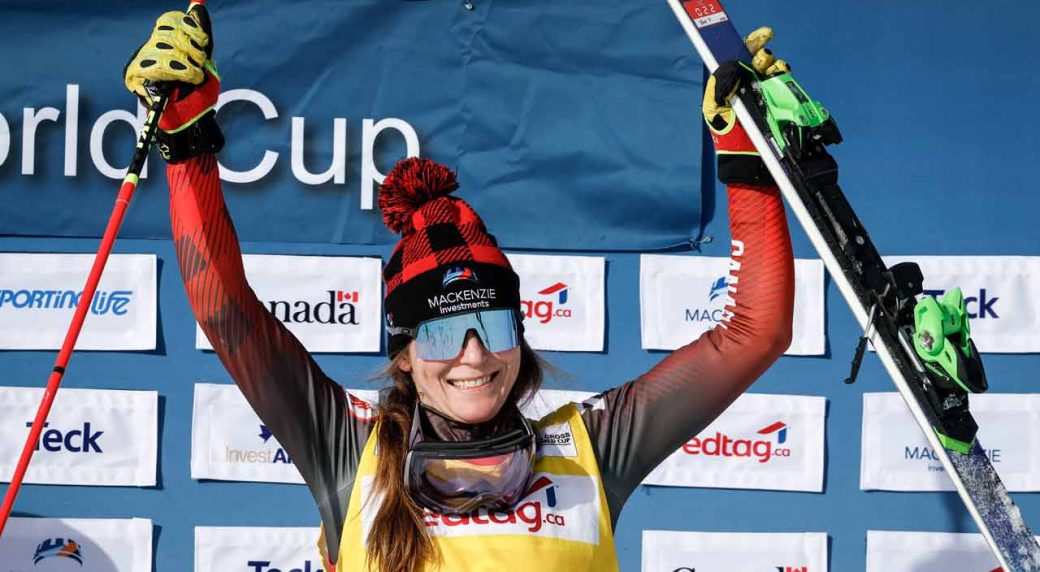This horizontal photograph captures a partial, angled view of a female skier posing in front of a blue vinyl sponsor banner adorned with various white squares and logos, including EdTag, Sporting Life, and the Country of Canada. She proudly raises a ski pole in her left hand and a ski in her right, with a beaming smile on her face. Her striking outfit features a red and black long-sleeve shirt topped with a bright yellow vest bearing an EdTag logo. She sports big thick yellow gloves, mirrored sunglasses, and a pair of ski goggles around her neck. Her distinctive red and black plaid beanie with a yarn pompom has "McKenzie Investments" emblazoned on the front. Her long brown hair is braided into a ponytail draped over one shoulder, adding to her dynamic and energetic appearance against the backdrop of the World Cup banner.